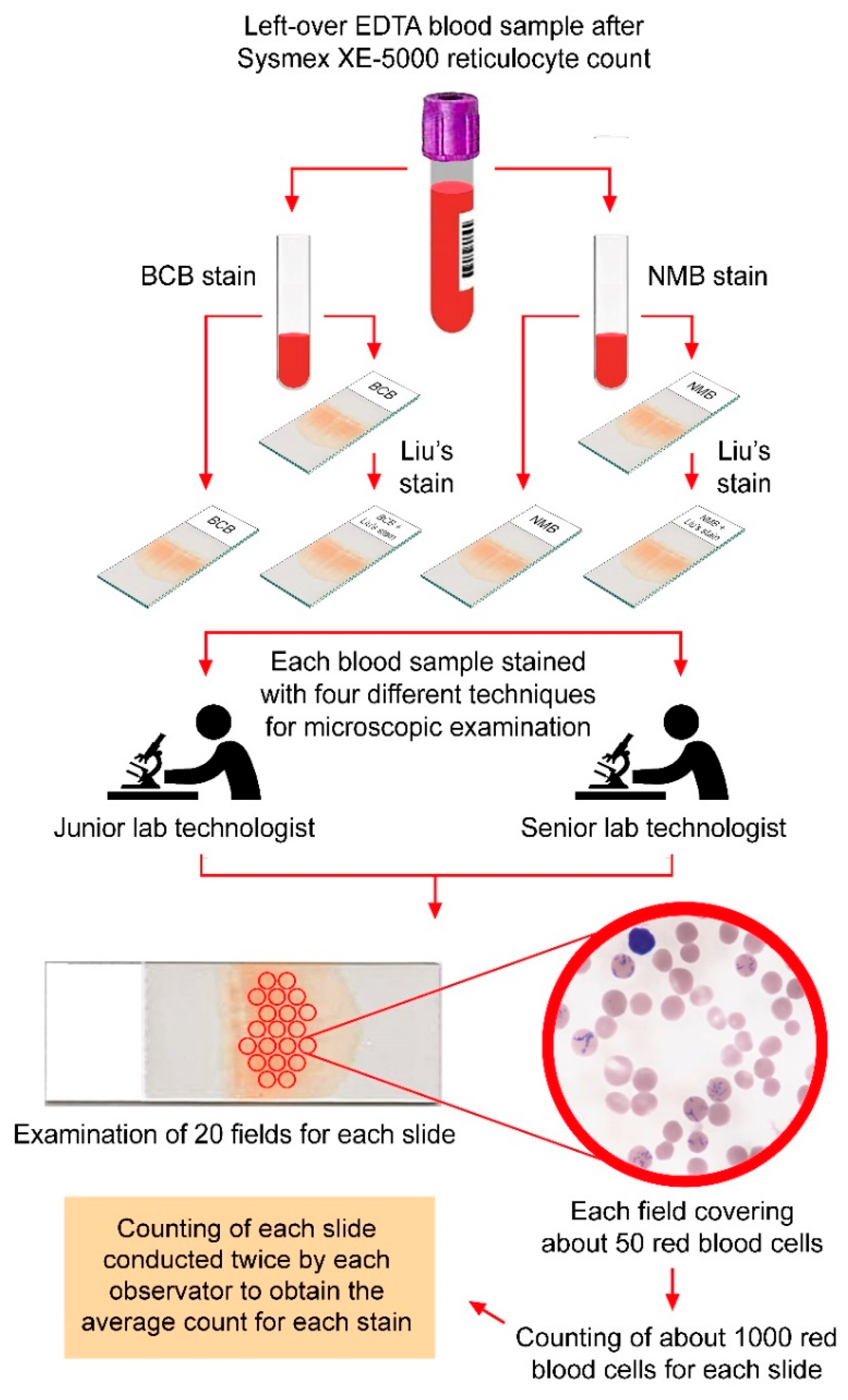This is a detailed digital diagram illustrating the process of examining a leftover EDTA blood sample after a Sysmex XE5000 reticulocyte count. At the top center of the diagram, the text reads "Leftover EDTA blood sample after Sysmex XE5000 reticulocyte count" in black. Below this, there is an image of a test tube containing a red liquid. The diagram then splits into two further test tubes, each representing different staining techniques. Moving downward, two rectangular sections detail staff involvement: one showing a junior lab technician and the other a senior lab technologist, both depicted in black line drawings without facial features, working with microscopes. Each blood sample is stained using four distinct techniques for microscopic examination, with text under each image explaining the process at each step. The arrows in the diagram, which are red, guide the viewer through the flow of the procedure. The background of the image is white, reinforcing the clarity and focus on the textual content and red directional arrows. The detailed method involves examining 20 fields for each slide and counting each slide twice by an observer to obtain an average count of the stain.